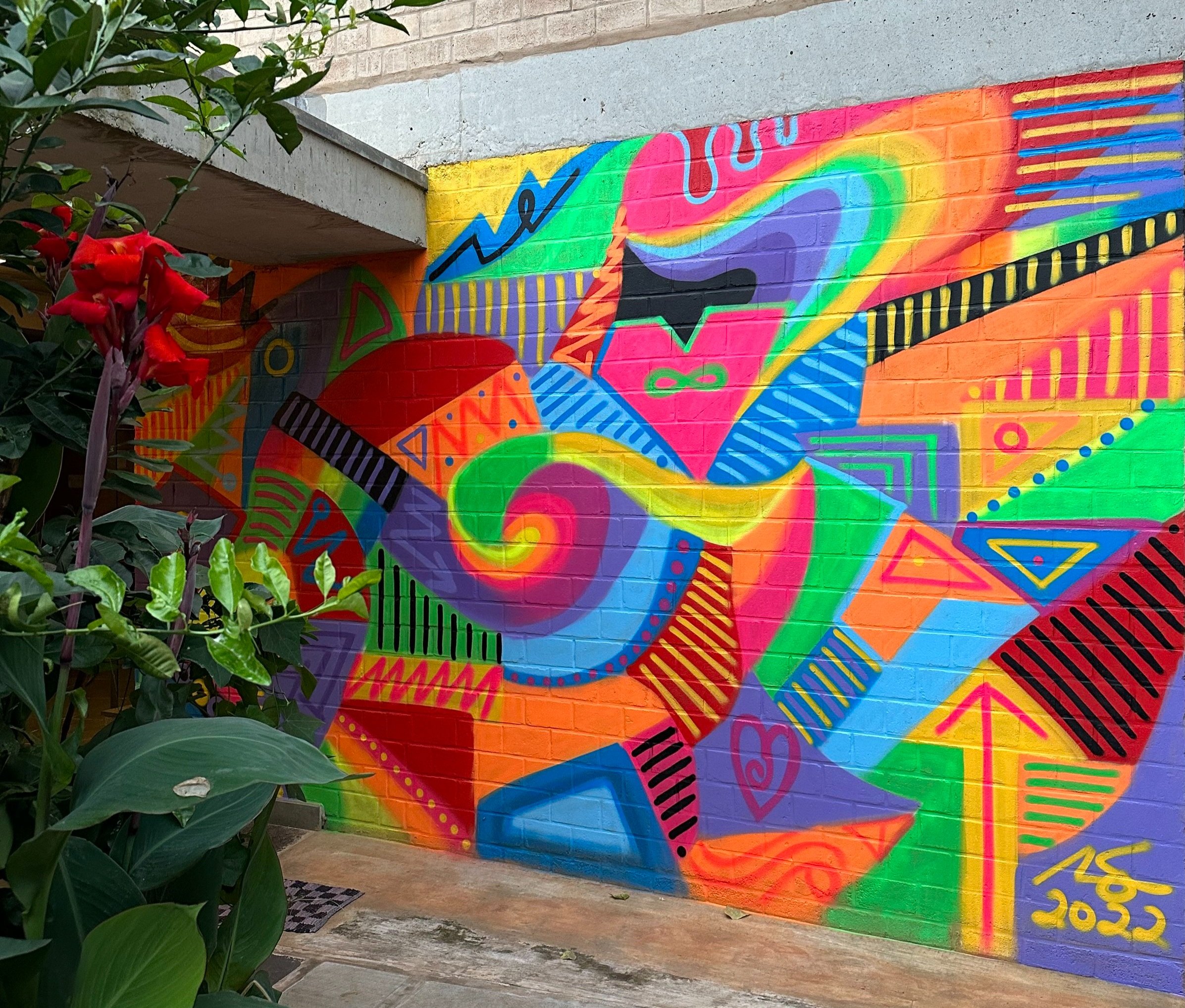The image showcases the vibrant side of a brick building adorned with a colorful, artistic mural painted graffiti-style. The mural features a stunning array of bright, vivid colors including black, red, blue, yellow, orange, pink, green, purple, and turquoise. The artwork is a dynamic mix of geometric shapes, swirls, striped lines, arrows, hearts, zigzags, and sections resembling swooping rainbows and abstract parrots. Notable elements include red arrows surrounded by yellow, blue-outlined red drops on a pink background, and flame-like forms with red and yellow hues. In the bottom right corner, the mural is signed "RS 2022" in gold spray paint. Additionally, large green tropical plants with bright red flowers, possibly hibiscus, are positioned in front of the wall, adding a natural contrast to the painted design. The top of the building remains unpainted brick, and the ground in front is concrete with a small roof cover jutting out from the building's side.